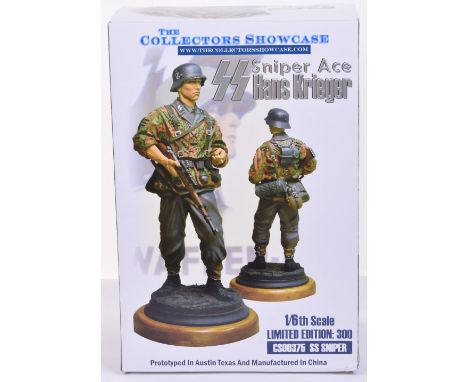The image depicts the outer cover of a collector's box for a detailed 1/6th scale limited edition action figure. The box displays two views of the figurine: a larger front view on the left and a smaller back view on the right. The action figure stands on a circular podium with golden and black colors. The figurine is dressed in a detailed army uniform, featuring a camouflage-colored jacket over a green-gray shirt, gray trousers, and black boots. The soldier is equipped with a rifle or gun and also wears a helmet, displaying a ready-for-combat stance. The front view shows the soldier looking to the right, while the back view reveals additional details such as a bag and supplies.

Text on the box includes "The Collector's Showcase" at the top in blue lettering. The right side reads "SS Sniper Ace, Hans Krieger," bearing the controversial double lightning bolt insignia of the SS. The bottom of the cover notes "1/6th scale, limited edition, 300," indicating the exclusivity of the item. Additional text specifies that the figurine was prototyped in Austin, Texas, and manufactured in China. The overall design highlights the military theme, targeted at collectors of detailed military figurines.